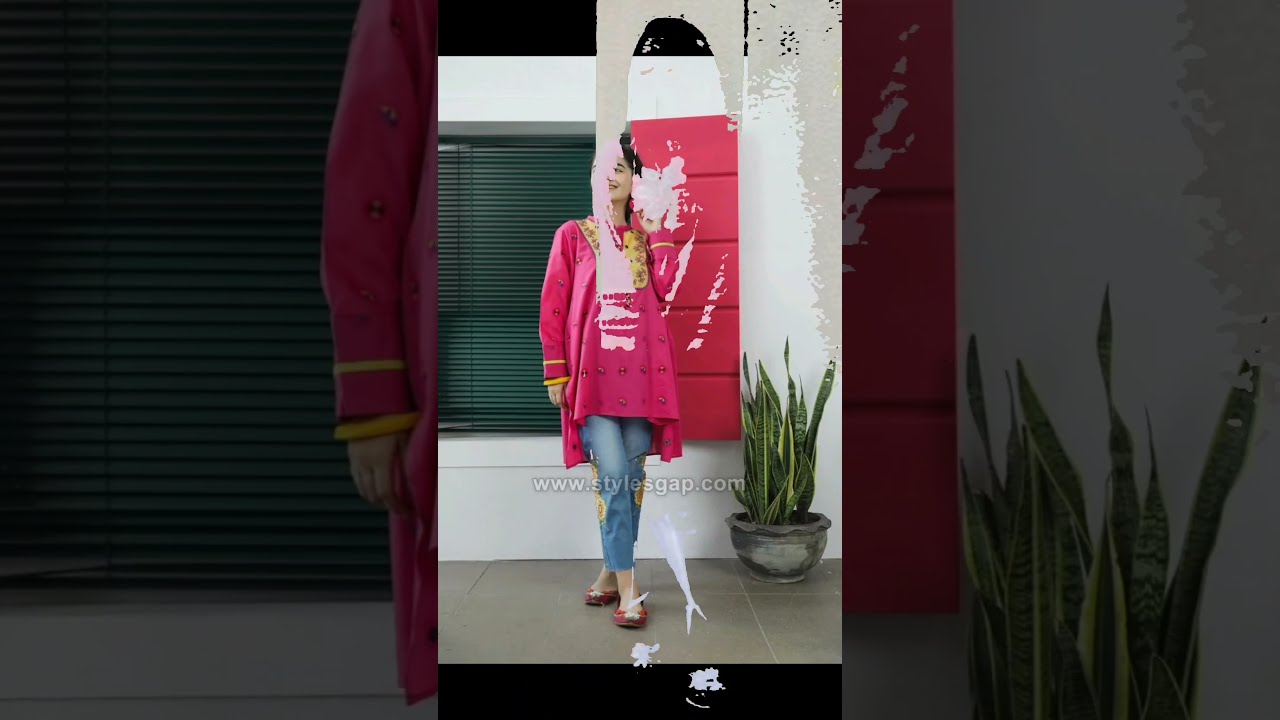The image features a young woman standing centrally, with a close-up of her left hand in the left third of the frame and a close-up of a wall with a black filter in the right third, which isn't very useful. The woman is positioned in front of a wall that has a window with green blinds and bright red shutters. She wears blue jeans paired with a unique pinkish-red coat/dress that has a longer back end, featuring a golden collar. The right sleeve appears yellow, adding a distinct contrast. She stands on a tile floor, with her legs crossed and her maroon slippers visible. There is a black pot with tall-bladed plants to the right of her, and above the window, the wall transitions to a grayish-white hue. The image is edited with brushstroke overlays that obscure part of her face, giving it an artistic touch. The text "www.stylesgap.com" is written across her knees in transparent white, suggesting the image is part of a fashion advertisement. The colors in the image include red, green, white, black, gray, yellow, gold, and brown. The various elements, including her attire and the window with its blinds and shutters, contribute to the detailed and fashion-forward atmosphere of the scene.